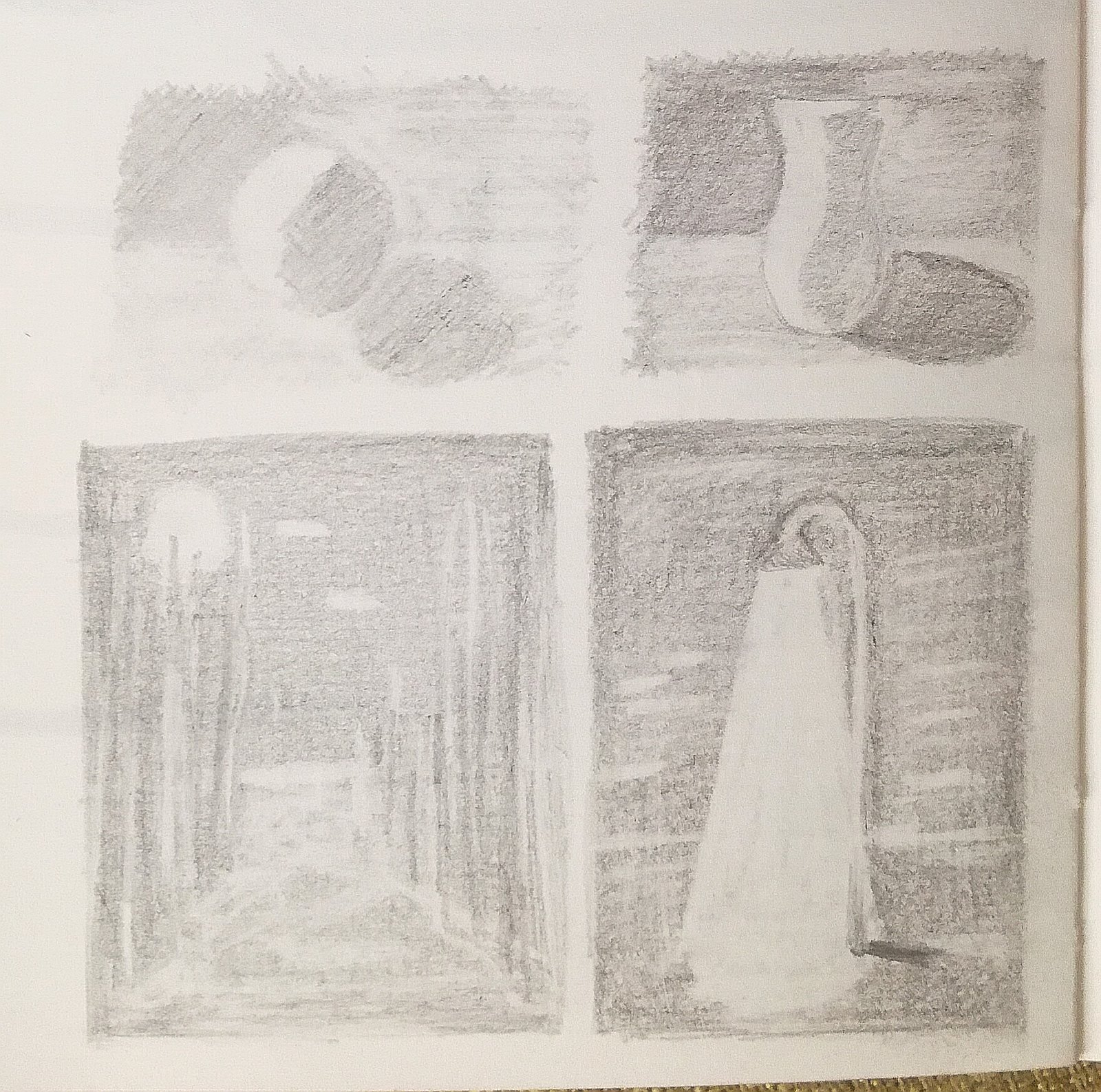The image showcases a large sheet of standard white artist's paper adorned with four meticulously shaded pencil drawings. 

In the top left corner, a rounded object—potentially spherical—features intricate shading on its right side, casting a corresponding shadow on the surface below. The background shading hints at a wall and table, providing context and depth.

Adjacent to this, in the top right corner, a darker-themed drawing depicts a vase. The right side of the vase is enveloped in shadow, with its form casting a distinct shadow onto the table beneath. Background shading enhances the scene's dimensional quality.

On the bottom left, a shaded pathway leads the eye through a serene landscape. Flanked by trees on both the left and right, the scene is enriched by distant clouds and a subtle hint of the sun, illustrating a tranquil outdoor environment.

Lastly, the bottom right drawing presents a lamp fixture, its origin—whether a streetlamp or an indoor light—ambiguity blending into the scene. The shading carefully differentiates the lamp's structure from the clear area where its light would emanate, creating a compelling interplay of light and shadow.